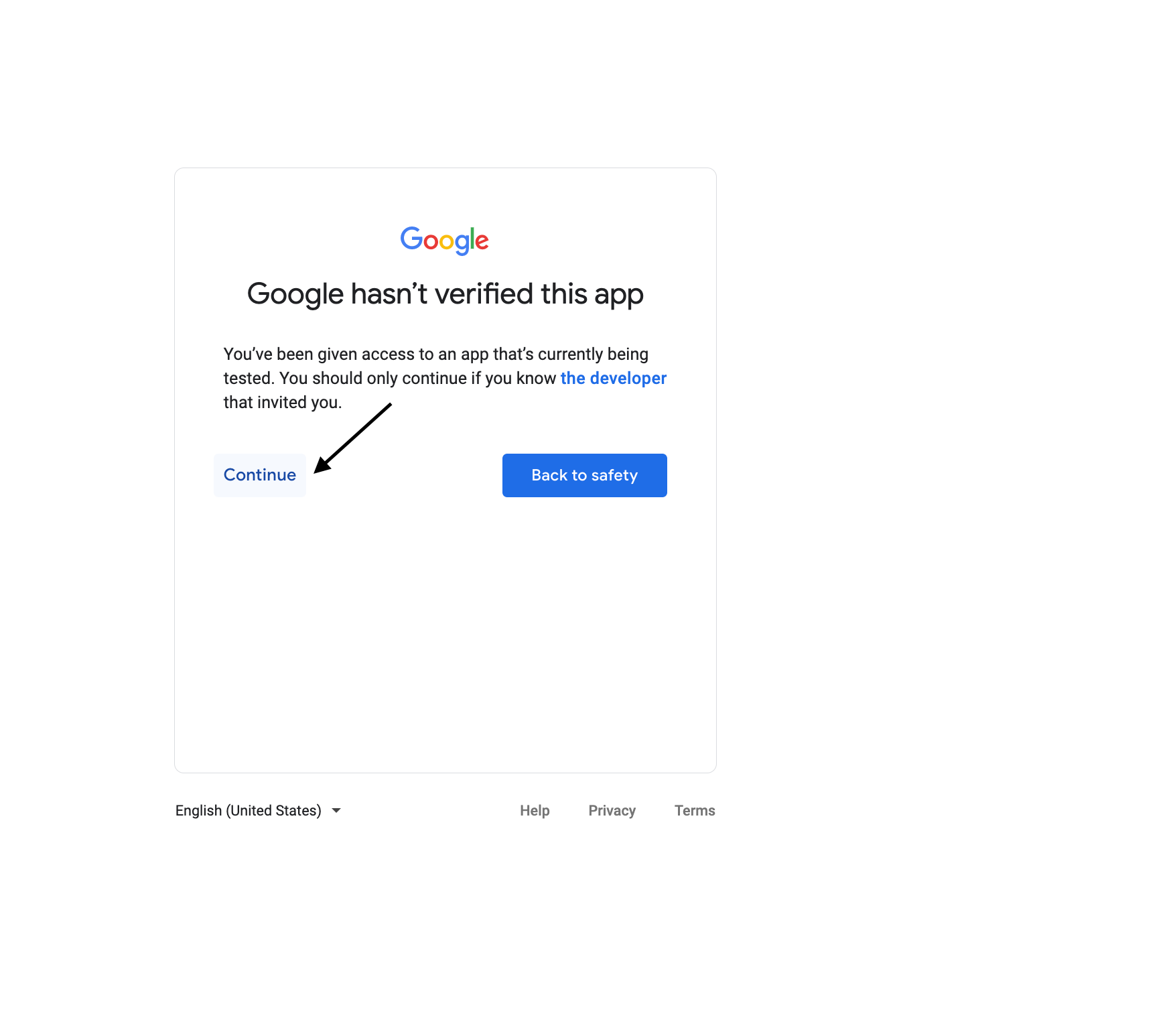The image depicts a Google pop-up notification, characterized by a grayish border with rounded corners. At the top center of the pop-up, the Google logo is prominently displayed, featuring its distinctive colors: blue, red, yellow, and green. Below the logo, in bold black text, the message "Google hasn't verified this app" stands out as the most prominent text on the page.

Underneath this headline, a smaller paragraph informs the user, in black text, that they have been given access to an app currently in the testing phase. The paragraph advises proceeding only if the user knows the developer, with "developer" highlighted in blue text for emphasis. An arrow extends from this paragraph, directing attention towards the bottom left of the pop-up.

In the bottom left corner, there is a gray button with blue text that reads "continue." In contrast, a blue button on the right-hand side features white text that says "back to safety." 

At the very bottom left, it reads "English (United States)," accompanied by a black arrow pointing downwards. The bottom right corner lists three links in gray text: "help," "privacy," and "terms." This overview encapsulates the detailed elements presented in the Google pop-up notification.